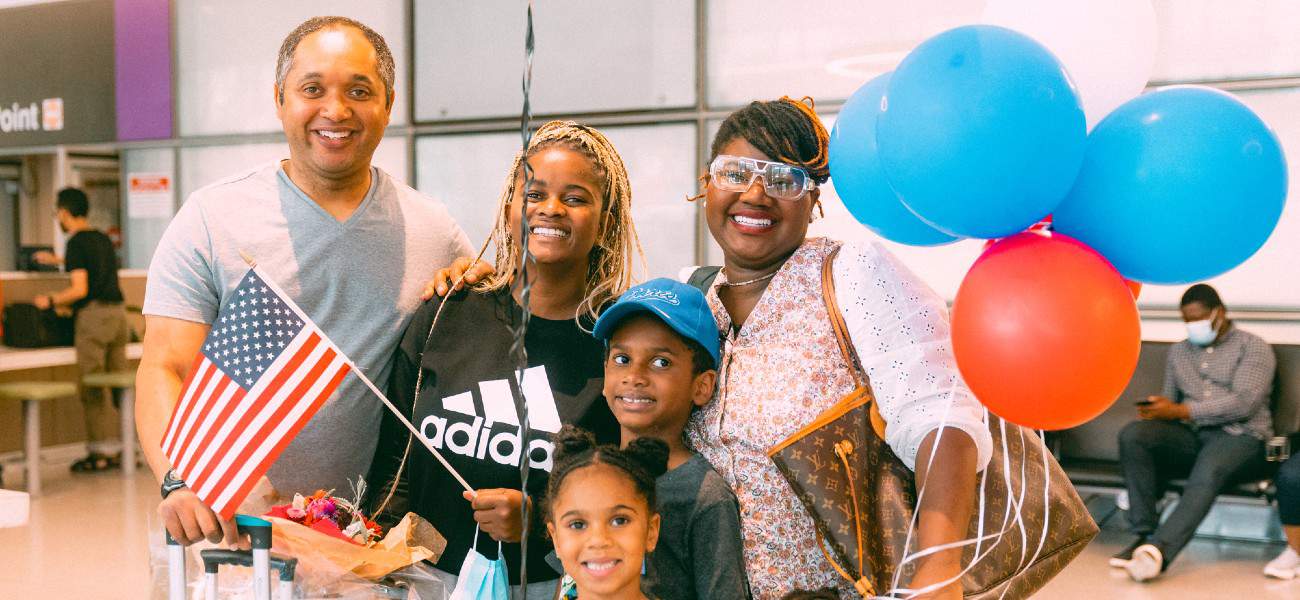This photograph captures a delighted African American family, likely comprising a father, mother, two daughters, and a son, all smiling broadly for the camera. The setting appears to be a public indoor space, probably an airport, suggested by the father's grip on a suitcase handle. Centered in the image is an older girl wearing a black Adidas sweatshirt and holding a small American flag and a surgical mask in her left hand. Next to her stands the father, dressed in a gray v-neck t-shirt. On the other side is the mother in glasses, a pink long-sleeved shirt, and a brown-and-orange leather handbag. She is holding a cluster of balloons—three blue and one red—suggesting a celebratory moment. The son, around eight or nine years old, stands between the mother and sister, sporting a blue ball cap and a green long-sleeved shirt with a tentative smile. Just below the son, peeking into the frame, is the youngest daughter with her hair in two buns and a charming smile. In the background, a man wearing a surgical mask sits on a black bench, emphasizing the public nature of the space. The entire scene exudes warmth and joy, potentially capturing a moment of arrival or reunion.